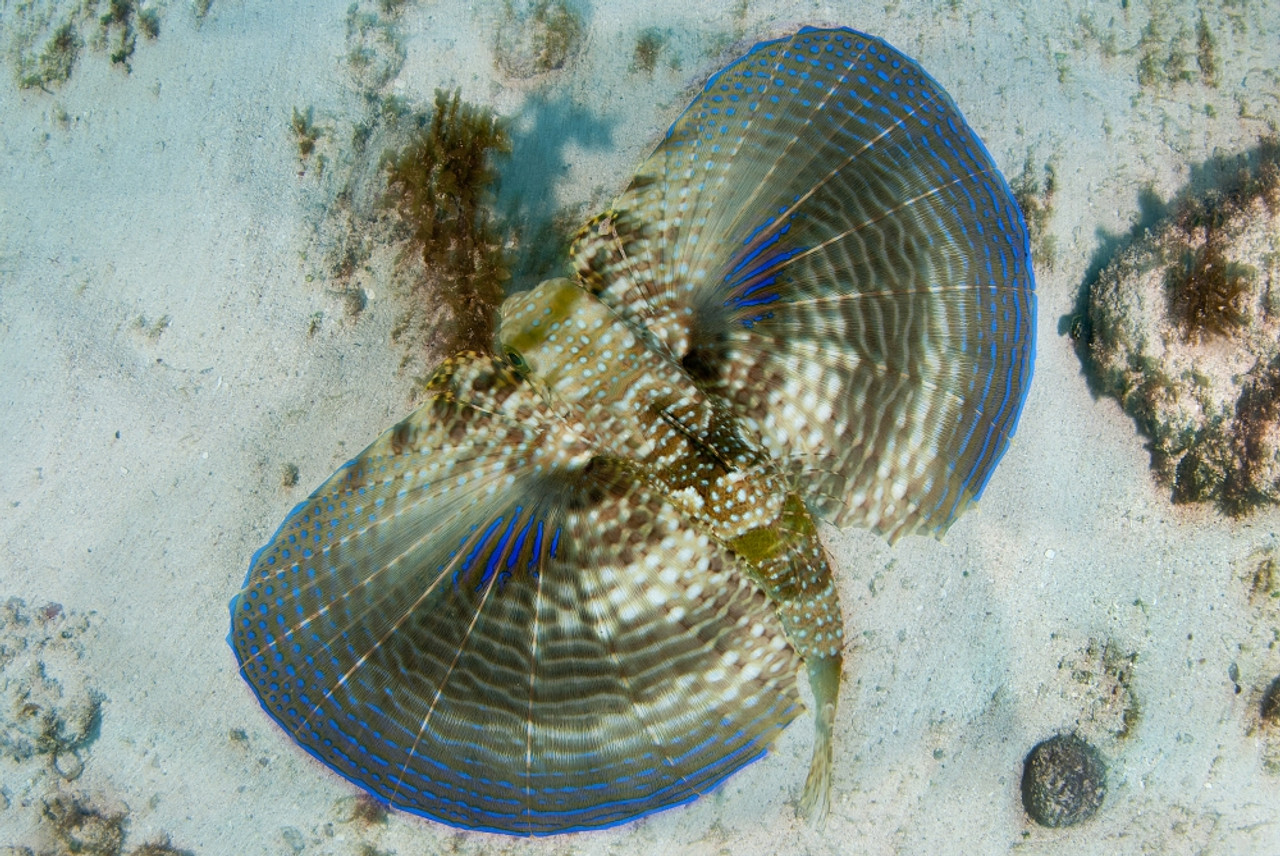This is a stunning color photograph of a fish, viewed from above, submerged in its natural underwater habitat. The fish, resembling a Clown Fish but not definitively identified, exhibits an exquisite display of color variations and patterns. Its gills are expanded, revealing a range of hues that include fluorescent blue edges, bands of beige and brown, and a captivating iridescent purple-blue spot. The fish's body is relatively short, adorned with a series of stripes and spots extending to its tail, which blend seamlessly into the surrounding terrain of the ocean floor, giving it a camouflaged appearance. Two prominent eyes are visible, suggesting the fish is being observed from a top-down perspective. The background is comprised of sea rocks, brownish-green seaweed, and sand, enhancing the natural beauty of the scene. Although the creature's wing-like extensions and intricate coloration lend it an almost abstract, butterfly-like appearance, the photograph clearly captures a moment of serene aquatic life.